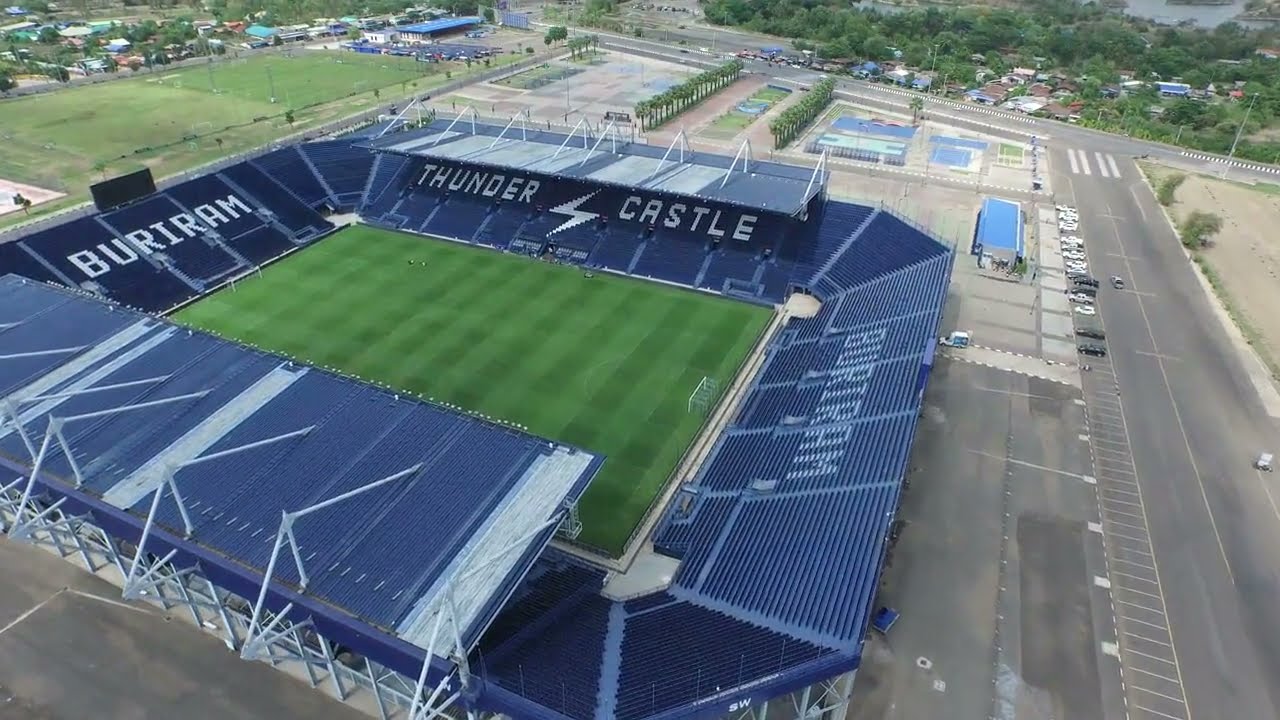The aerial view captures an empty soccer stadium with dark blue seats and a green field laid out in a grid pattern of light and dark green. White lettering on the seats spells out "Buri Ram" on the upper left and bottom right sections, and "Thunder Castle" on the upper right, complete with a lightning bolt between the words. Above "Thunder Castle," there is an awning supported by white metal pillars. The pristine field is clearly well-maintained, featuring white metal goals at either end. 

Surrounding the stadium is a concrete and asphalt parking lot, with about 20 vehicles scattered throughout, predominantly white. A two-lane street runs along the far right side, with a few cars driving and others parked in designated spots. The background scenery includes lines of trees running vertically and several open grassy fields, tennis courts on both sides, and a mix of houses interspersed among lush vegetation.